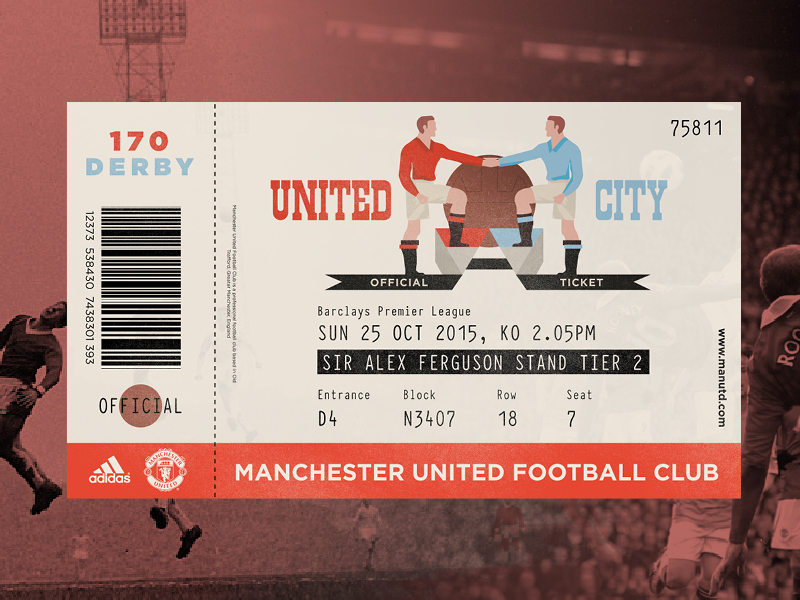This image features an official ticket stub for a match in the Barclays Premier League between Manchester United and Manchester City, held on Sunday, October 25, 2015, at 2:05 p.m. The ticket grants entrance through D4 to the Sir Alex Ferguson stand, tier 2, specifically for block N3407, row 18, seat 7. This event is billed as the 170th Derby, prominently displayed in red and blue. Notably, the ticket is identified with the number 75811 and includes the main sponsors' logos, Adidas and the Manchester United Football Club crest. Additionally, the URL www.manutd.com is listed on the ticket. The background of the ticket displays an engaging scene of the stadium, featuring a drawing of two football players, one in a red jersey, representing United, and the other in a blue jersey, representing City, shaking hands, symbolizing sportsmanship.